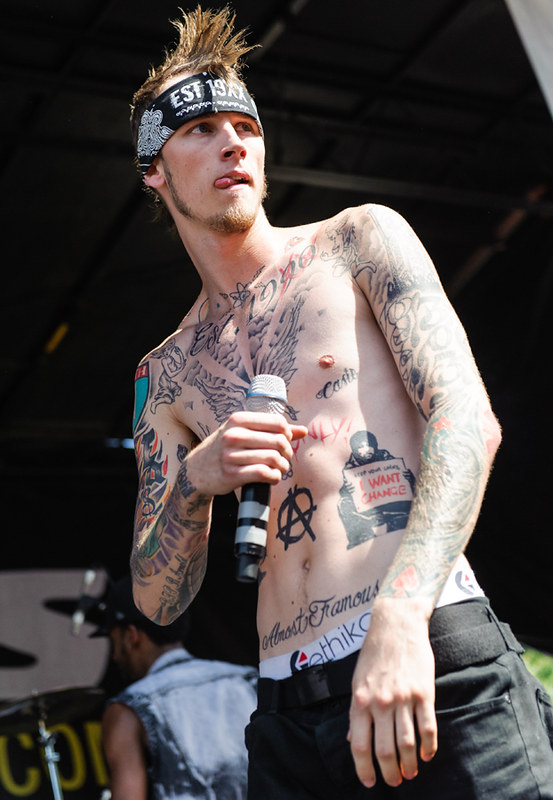In this picture, the scene is set on a high-ceiling stage with visible rafters at the top. The main focus is a shirtless male figure prominently centered in the photo, slightly tilted to his right, possibly due to the camera angle. He sports a medium brown faux-hawk hairstyle and wears a black headband with white lettering that reads "EST 19XX." His tongue is out, and his mouth is slightly open, suggesting he is in the midst of performing or about to speak. Covering his chest and arms are numerous tattoos, including legible words on his stomach and a blue shield tattoo on his right shoulder. Clad in black pants with a black belt, he holds a microphone in his right hand, his right elbow bent. In the background, another male figure can be seen facing away, dressed in a blue jean jacket, adding depth to the scene.